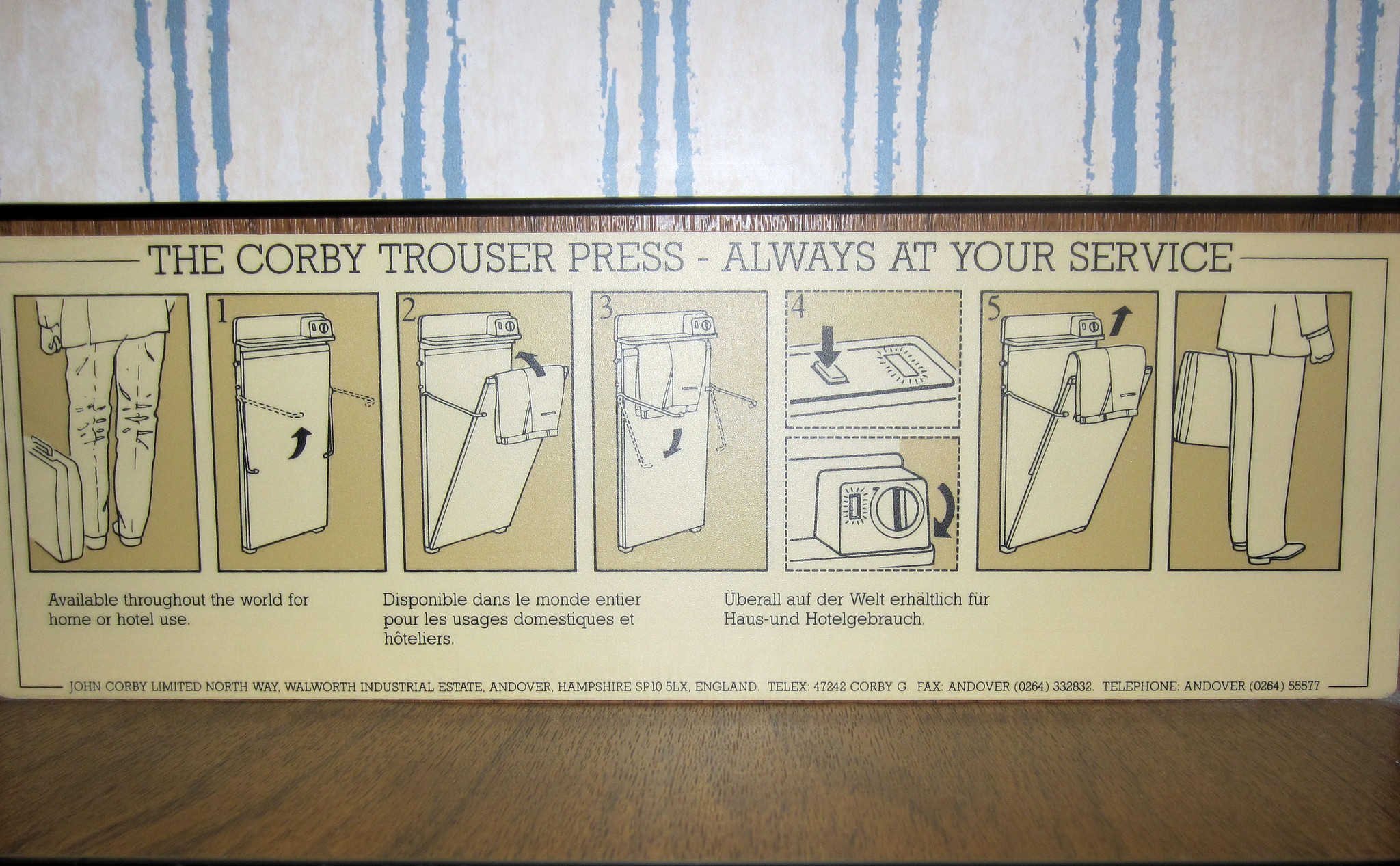The image showcases a detailed and instructional diagram displayed within a picture frame. The focal point of the image is the Corby Trouser Press, prominently labeled with the phrase "The Corby Trouser Press - Always at your service." The diagram is sectioned into six distinct squares, each depicting step-by-step photographic instructions on how to effectively use the trouser press to press pants. Below these six instructional squares, a message states: "Available throughout the world for home or hotel use," which is reiterated in two additional languages, emphasizing the product's global availability.

At the very bottom of the image, contact information for John Corby Limited is provided. The address listed is Northway, Walworth Industrial Estate, Andover, Hampshire, SP10 5LX, England. The contact details include a telex number: 47842 Corby G, a fax number: 0264 332832, and a telephone number: 0264 555577.